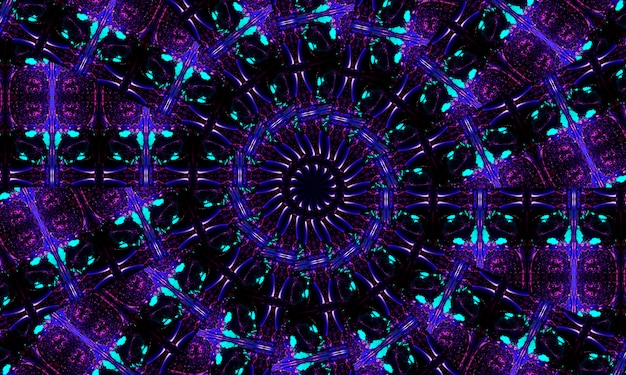This abstract, computer-generated artwork features a highly intricate, circular pattern composed of multiple symmetrical layers, drawing the viewer's gaze towards a central point. The image is characterized by an array of geometric shapes, including rectangular segments and thinner lines extending outward in a sort of X-shape from the center. The color palette transitions fluidly between rings, starting with black, shifting to a circular arrangement of light purple stripes, then alternating back to black, and evolving through gradients of light to dark purple, pink, and teal, with hints of blue and light pink interspersed. Some sections resemble pods that radiate from the inner circle, combining to create a compelling, pronged structure. Although the artwork captures part of a larger circle within a square frame, it maintains a complex and mesmerizing symmetry that features contrasting colors such as black and green prongs, with adjacent sections in shades of gray and pink, adding to its intricate visual appeal.